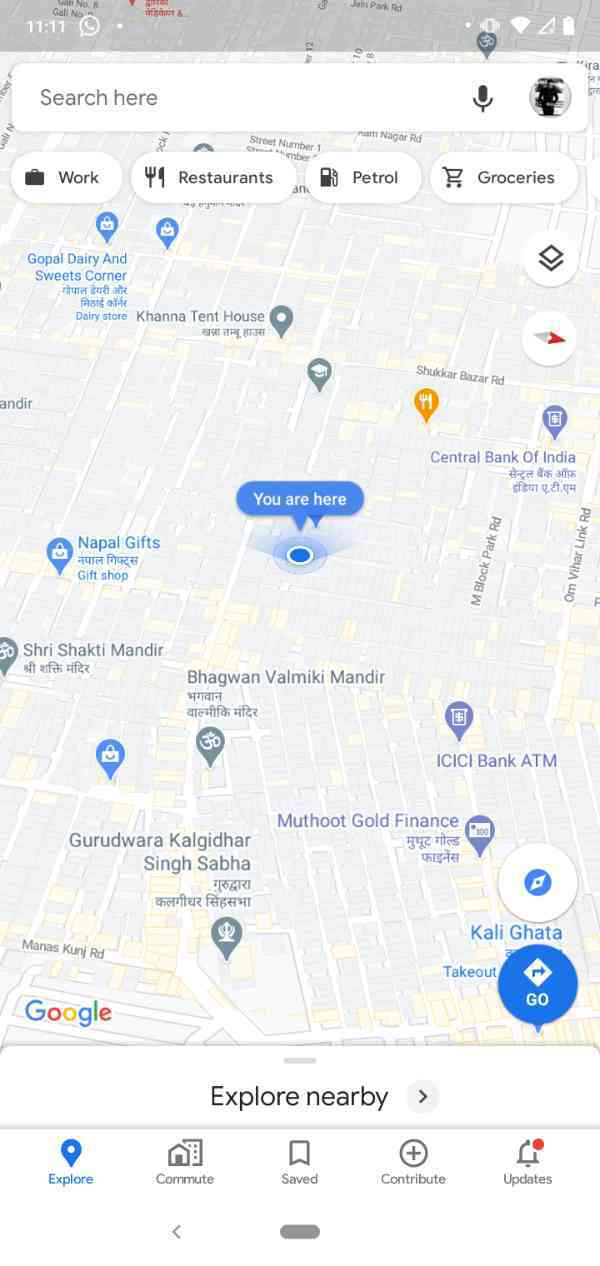The top of the display shows the time as 11:11. Below the time is a long rectangular search bar labeled "Search here." To the right of the search bar, there's an icon of a microphone, allowing users to activate voice search. Below the search bar, the word "Work" appears, followed by categories labeled "Restaurants," "Petrol," and "Groceries," all of which are centered around a map.

On the map, various locations are marked by blue circles with icons indicating their types. There is one location labeled "Dairy and Sweets Corner." At the center of the map, a marker indicates "You are here." To the left of this central marker, another blue circle denotes "Nepal Gifts Gift Shop." To the right, an orange circle with a fork and spoon icon might represent a restaurant.

Toward the bottom of the map, an "ICI Bank ATM" is listed, alongside "MUT HOOT Gold Finance" marked with a purple symbol and a white square. At the very bottom, there's a prompt to "Explore nearby."